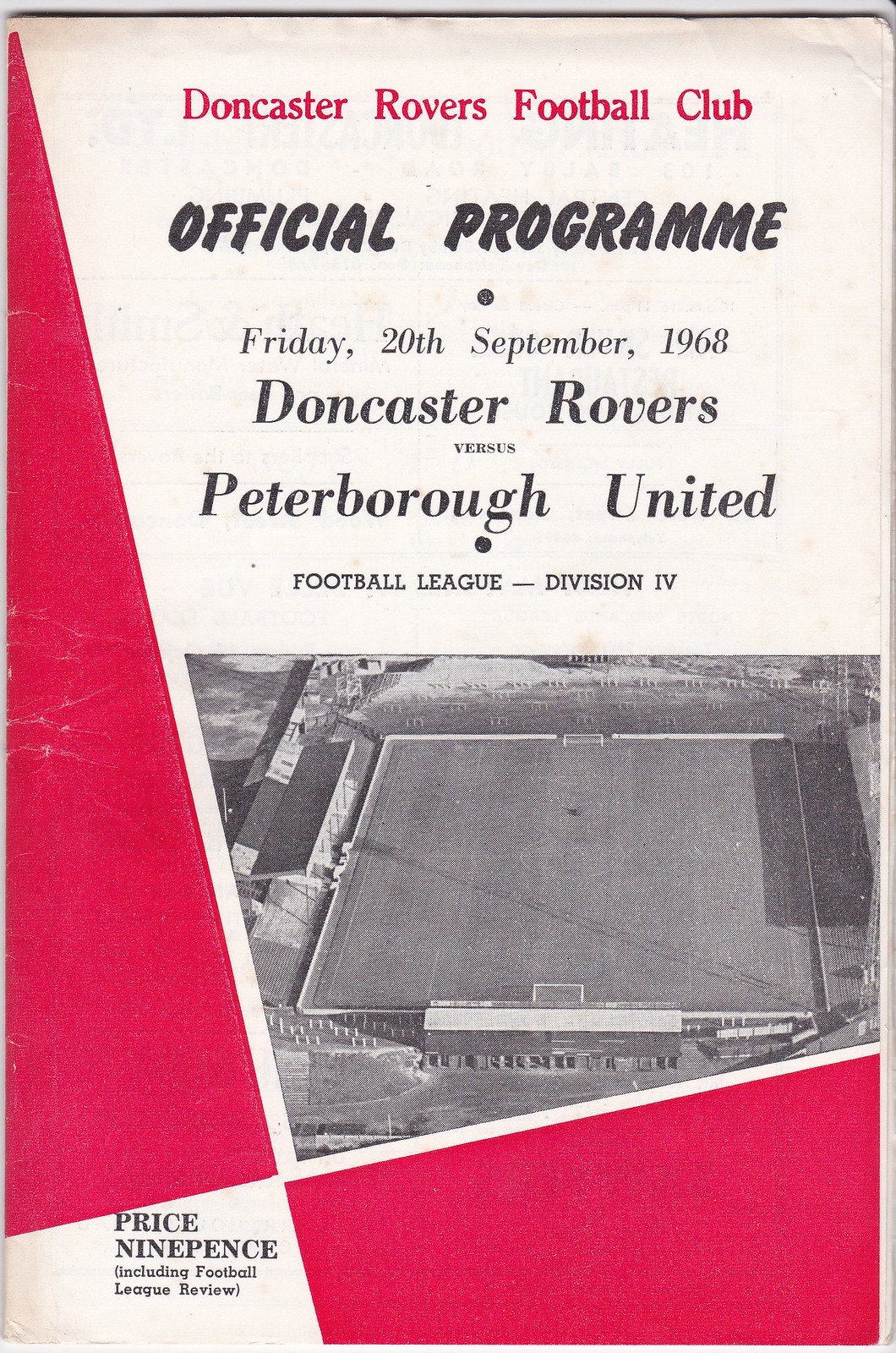The image is a vertically aligned rectangular picture of the front cover of a worn football program booklet. The top section is light gray or white, with visible wrinkles along the top and along the left edge where the spine is. Prominently displayed in the center at the top, in red letters, is the text "Doncaster Rovers Football Club". Below this, in all caps black letters, it reads "Official Program". Underneath is a small circular dot, followed by the date "Friday 20th September 1968". Further down, it says "Doncaster Rovers" in smaller letters, followed by "Versus" and then "Peterborough United". Another black dot follows this information, leading to the text "Football League - Division IV".

In the middle of the cover, there is a black and white aerial photograph of an empty, square soccer field, complete with visible goal posts and white nets. To the right of the photo, there is a large, solid red triangular section, with a trapezoidal red section beneath it. 

In the lower left-hand corner, the price is listed as "Price Ninepence", and in small print beneath it, it states "Including Football League Review" in parentheses.

This detailed description captures the shared and repeated elements provided by the two original captions, blending them into a unified, thorough depiction of the image.